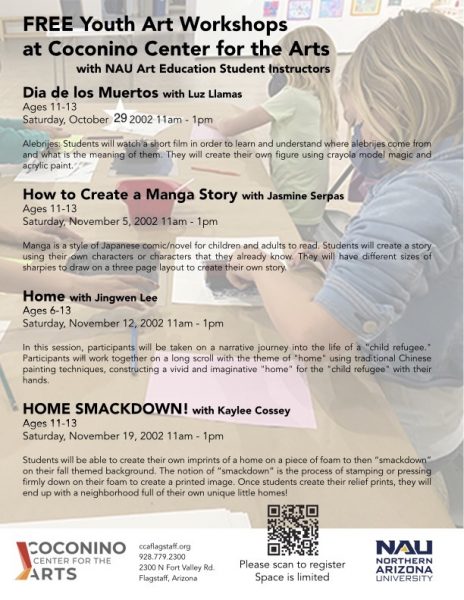This flyer advertises free youth art workshops at the Coconino Center for the Arts, in collaboration with Northern Arizona University (NAU) Art Education Student Instructors. In bold letters at the top, it announces the event, with a captivating background image of young children engaged in art activities. Below, it details four upcoming workshops:

1. **Dia de los Muertos with Luz Llamas**: Participants will watch a short film to learn about Alebrijes, their origins, and meanings. They will then create their own figures using Crayola Model Magic and acrylic paint.
2. **How to Create a Manga Story with Jasmine Serpas**: A creative session focused on crafting manga narratives.
3. **Home with Jingwen Li**: This workshop takes participants on a narrative journey of a child refugee’s life. They will collaboratively create a scroll themed around home, using traditional Chinese painting techniques.
4. **Home Smackdown with Kaylee Cossie**: Attendees will design and imprint home-related pieces on foam, which will then be pressed onto fall-themed backgrounds.

The flyer highlights essential information at the bottom, including the Coconino Center for the Arts logo, location details, a QR code, and the NAU logo.